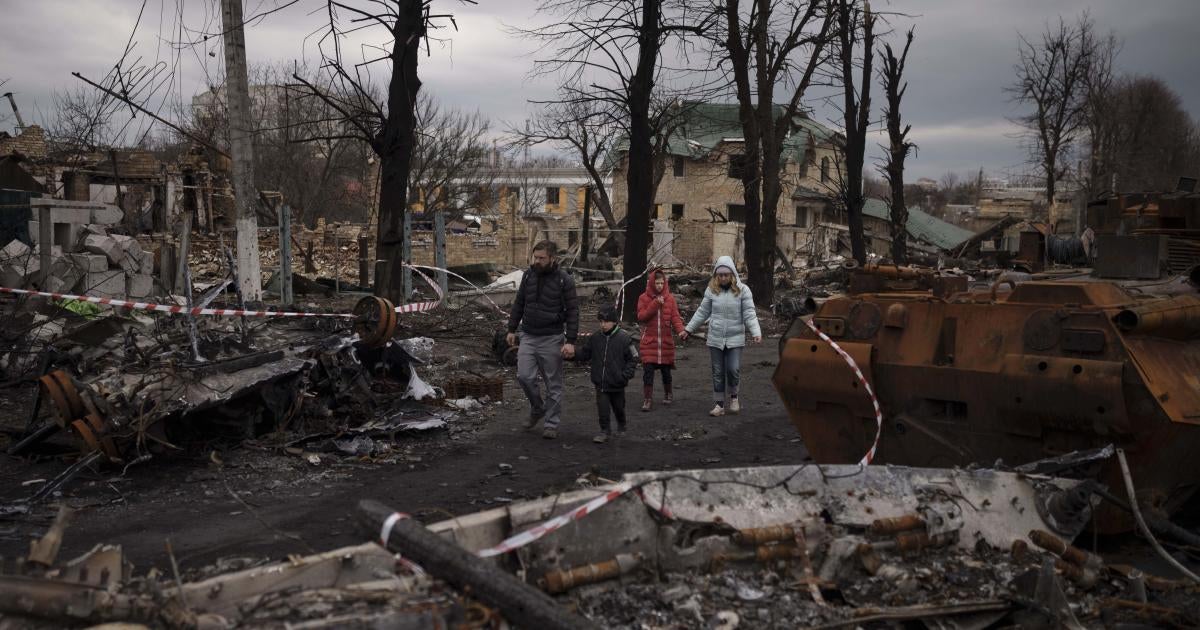The image captures a somber scene of destruction, set in a town that has been ravaged, possibly by a tornado or an attack. Debris and wreckage are scattered everywhere, with several buildings reduced to rubble. Red and white caution tape flutters in the wind, partly displaced, hinting at a recent catastrophe. The sky is a bleak gray, the overcast clouds enhancing the gloomy atmosphere. In the background, dark, leafless trees, some appearing burnt, stand like silent witnesses to the calamity. 

Amidst this desolation, four figures traverse the devastated landscape. Leading the way is a man in a black jacket and gray pants, firmly holding the hand of a young boy who is dressed in all black and wearing a hat. Following closely are a woman in a white jacket, blue pants, and white shoes, walking hand-in-hand with a girl clad in a red jacket and black pants. The group moves cautiously through the rubble, their coats and demeanor reflecting the cold and dismal environment. 

To the side, remnants of metal and other wreckage lie about, adding to the chaotic setting. Despite the destruction around them, the group remains closely bonded, navigating through what was once a normal town now left in ruins.